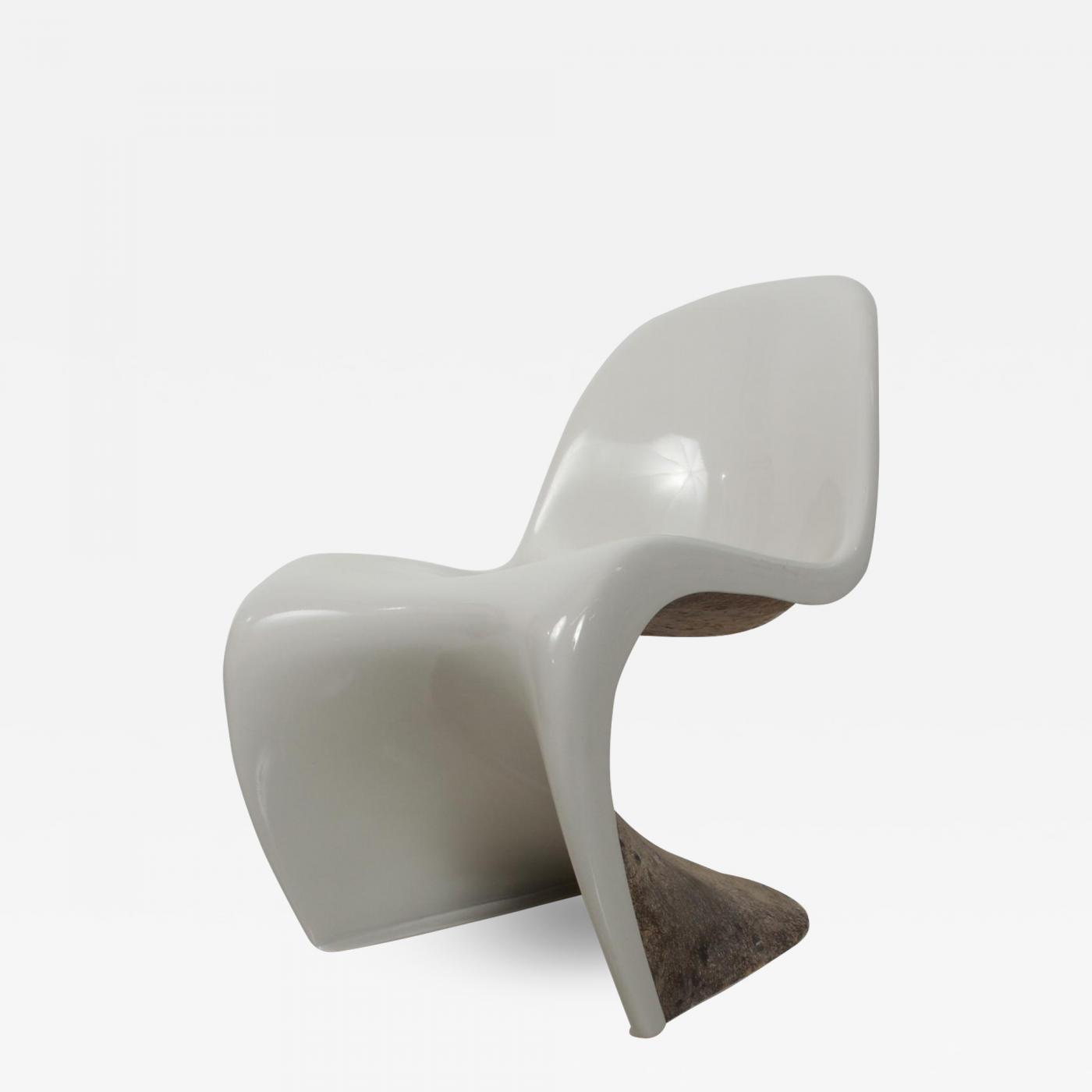This photograph showcases an intriguing, abstractly designed chair that resembles a modern art sculpture. The chair is crafted from what appears to be a single, continuous piece of material—potentially wood with a glossy white finish on the surface. The front is shiny white, while the back displays a brownish or darker gray hue, possibly resembling wood grain. The chair's form is highly irregular and contoured, featuring a curvaceous shape that twists elegantly to create both the seat and the backrest. This design incorporates a bucket-like seat with recessed areas for comfort. The chair lacks traditional legs, instead resting on a concave, horseshoe-shaped base that provides support. Its unique aesthetic evokes a mid-century modern or futuristic style, likely making it a valuable yet potentially impractical art piece.